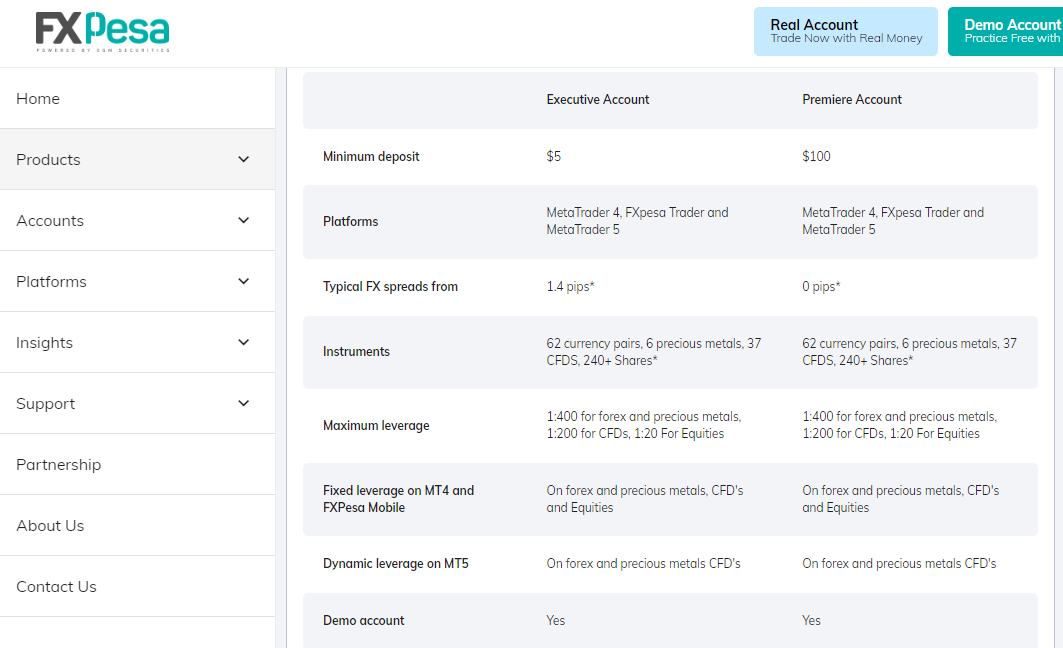The digital image is a screenshot from the FXPesa website, showcasing different account options available for trading. The site offers the flexibility to trade with real money through a "Real Account" or practice trading skills using a "Demo Account," free of charge. Two account types are available: the Executive Account, requiring a minimum deposit of $5, and the Premier Account, which necessitates a $100 minimum deposit.

The image lists various trading platforms supported by FXPesa, including MetaTrader4, FXPesaTrader, and MetaTrader5. It also highlights the range of tradeable instruments, including 62 currency pairs, 6 precious metals, 37 CFDs, and over 240 shares. The platform offers dynamic leverage on MT5 for forex and precious metal CFDs.

The left side of the image features a navigation menu with buttons for Home, Products, Accounts, Platforms, Insights, Support, Partnership, About Us, and Contact Us, providing easy access to different sections of the website.